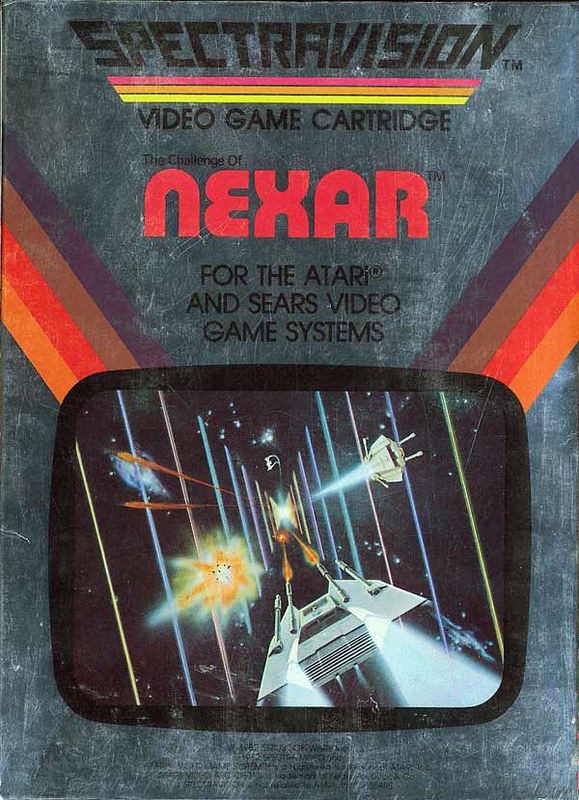The image features a vintage video game cartridge titled "The Challenge of Nexar" designed for the Atari and Sears video game systems. The cartridge is branded with the SpectraVision logo at the top. The label beneath the logo showcases a dynamic out-in-space theme, flanked by vibrant, cartoonish multicolored ribbons on each side, adding a playful aesthetic. The title, "The Challenge of Nexar," is prominently displayed in the center against the cosmic backdrop. Below the title, there is a descriptive stripe in pink, orange, and yellow, reading "Video Game Cartridge." The background of the cartridge label mimics a grayish stone texture, interspersed with white areas, enhancing its vintage appeal. Small, illegible text is located at the bottom of the packaging, contributing to the overall antique look.